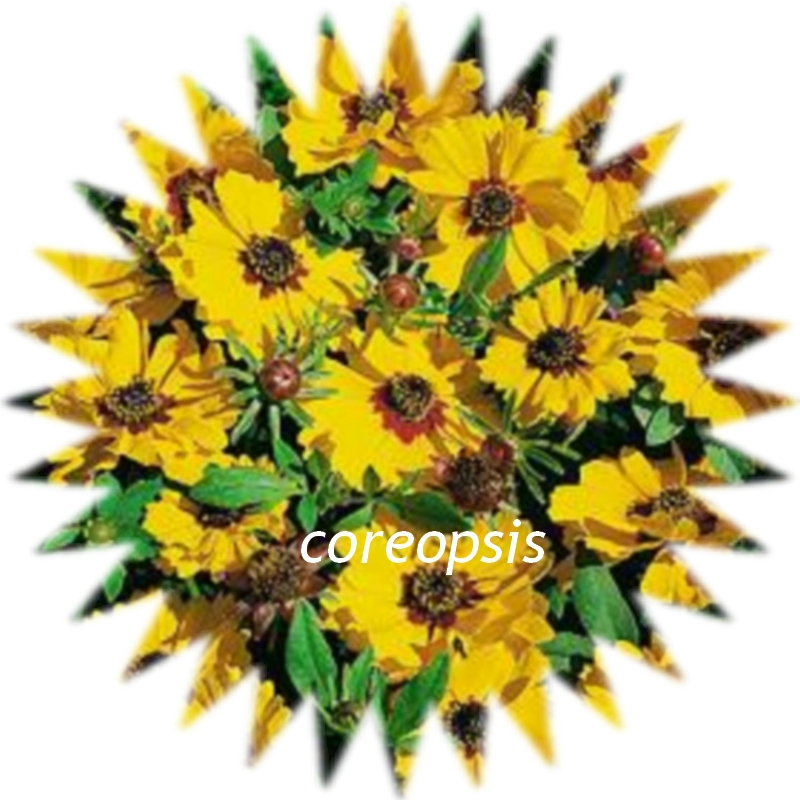The image features a graphic depiction of several bright yellow flowers, resembling marigolds, arranged in a circular, sun-like pattern with triangular spikes or rays emanating outwards. These rays are predominantly green, with hints of yellow, brown, and black, creating a vibrant and textured appearance. The flowers boast large yellow petals with a central core that appears brownish-red, tapering to black at the center. Interspersed among the flowers are small green leaves and a few closed buds resembling reddish-brown buttons. The background is a solid white, enhancing the contrast and vividness of the floral arrangement. At the bottom of the image, white text spells out "Coreopsis," identifying the flowers' scientific name.